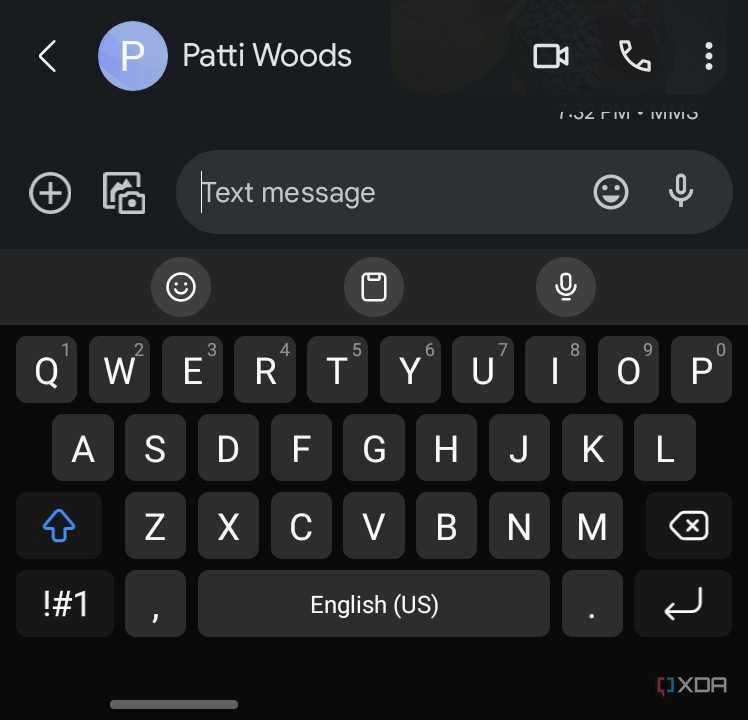The image depicts a detailed view of a messaging interface on a mobile phone. At the top, there's a blue sticker featuring the letter 'P'. Below this, the name "Patty Woods" is prominently displayed. Adjacent to this, two icons are visible—one resembling a video camera and another resembling a telephone. A vertical line of three white dots follows, and beneath them is a circular button with a plus sign inside it. Another icon appears next to this arrangement.

Further down, there's a text input field marked "text message," featuring both a smiley face icon and a microphone icon within the same area. The lower section of the image reveals a virtual keypad. The top row of this keypad displays letters, each paired with corresponding numbers from 1 to 0. All characters are in white print, with the exception of the 'up arrow' key, which is highlighted in blue to stand out from the rest. Additionally, there's a visible return button for sending messages or creating line breaks.